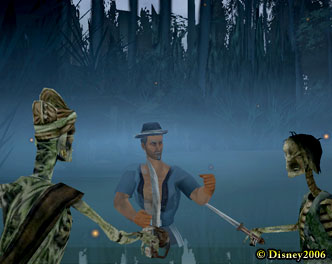The screenshot from a Disney production dated 2006, evident from the yellow copyright symbol in the lower right corner, presents a vivid scene rendered in a blue-tinted, fog-like atmosphere. In the background, tall tree trunks emerge, fading into the misty blue fog. The foreground captures a dramatic encounter: two skeletons positioned to the left and right, visible from the mid-torso upwards, engage in combat. The skeleton on the left dons a gray hat, while its counterpart on the right wears a black hat. Centrally framed, a muscular cartoon man, wearing a fedora, fiercely battles the skeletal figures, highlighting the scene's intensity and animated style.